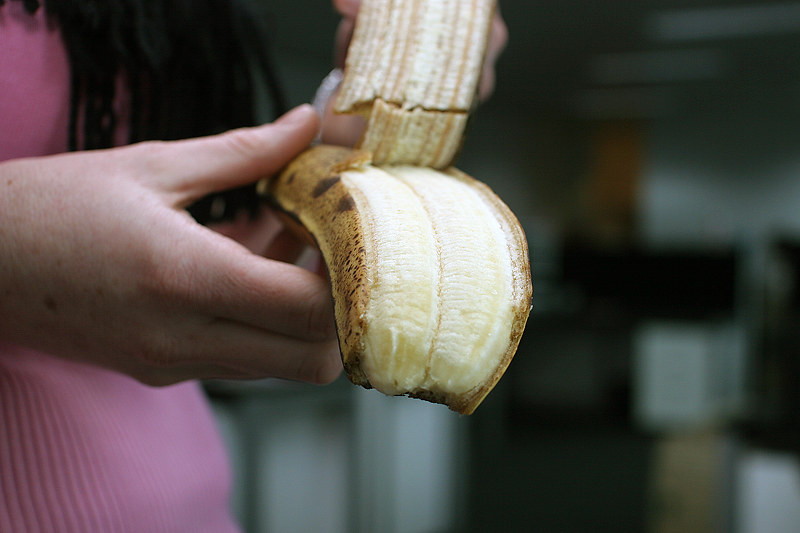In this image, a person, partially out of focus and positioned to the left, is holding a ripe banana in their right hand. The person's distinct, pink ribbed shirt stands out, while their hand and the banana are the primary focal points. They are in the process of peeling the banana, with one section already pulled back, revealing a crack across that part of the peel. The banana itself displays signs of ripeness, with its deep yellow skin adorned with brown spots and some black markings near the top where the peeling begins. The fruit has a prominent downward curve. The blurred background features dark colors, including possible shades of green and black, adding depth to the overall composition.